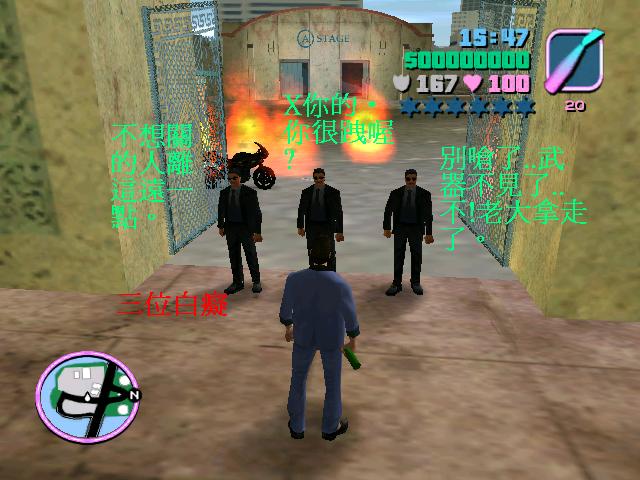This image is a brightly-colored screenshot of what appears to be Grand Theft Auto: Vice City, given the indicative vibrant blues and greens. It features a scene set in a street or alleyway, possibly a studio film lot, with three men in dark suits and sunglasses blocking a gate with the word "STAGE" over the two large doors behind them. The main character, dressed in a blue suit, is positioned in front of the trio, holding a Molotov cocktail.

The upper right corner of the image displays various game statistics, including the time stamp "1547," a financial standing of "five billion dollars" represented as the number 5 followed by roughly 8 or 9 zeros, a shield rating of 167, a heart rating of 100, and zero stars. There is also a pink and blue line with a "20" underneath it, and the text is primarily in Chinese characters written in light green. The bottom left corner showcases a map, likely indicating the player's current location within the game.